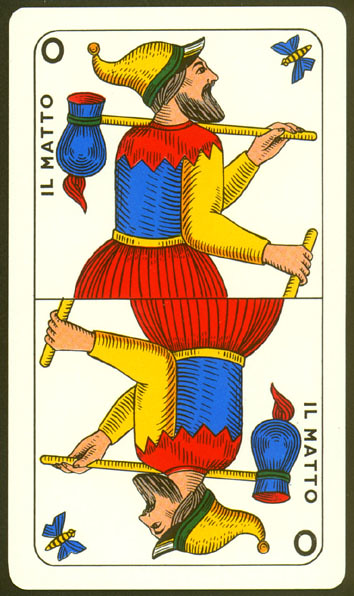This image features a distinctive cartoon character, likely from a playing card, with a mirrored counterpart below, indicating the card's dual orientation. The card is outlined in black and has a white background. At the top of the card, the word "Yomato" is prominently displayed, suggesting a different language or a specific title. A zero is placed in the top left corner of the square, while in the top right corner, a bee-like insect with a yellow body, black stripes, and blue wings hovers.

The central figure, a whimsical man, carries a stick over his shoulder with a blue and red bundle, reminiscent of a hobo's bindle. He sports a yellow and green hat, resembling either a pajama cap or a court jester's hat, and his multi-colored outfit includes a red upper section, a predominantly blue torso, and yellow sleeves. His right hand holds another stick pointed downward.

The bottom half of the image mirrors the top exactly, with the character now facing the opposite direction, reinforcing the symmetry typical of playing cards. The mirrored bee appears in the bottom left corner, aligned with the upside-down version of the man, who now faces left.